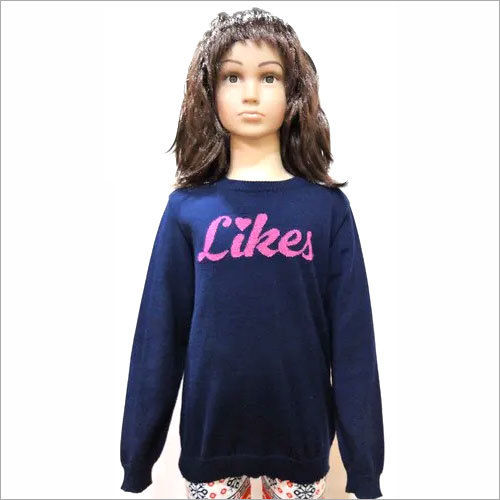Centered against a stark white background framed in black, the image features a mannequin with a stylized, life-like face and deep brown eyes. The mannequin, resembling a female figure with long brunette hair cascading to its shoulders, has an expressionless stare. It is dressed in a deep blue, long-sleeved sweatshirt adorned with cuffed sleeves, a cuffed bottom, and a cuffed neckline. Across the front of the sweatshirt is the word "LIKES" written in pink cursive lettering, with a heart-shaped dot over the 'i'. The mannequin's lower half is outfitted in patterned pants, decorated with snowflake designs interspersed with small orange diamonds. The overall setting is ambiguous, possibly depicting either a child's bedroom or a mannequin in a storefront display. The image is characterized by the contrast between the mannequin's detailed attire and the expansive, unadorned white space surrounding it.